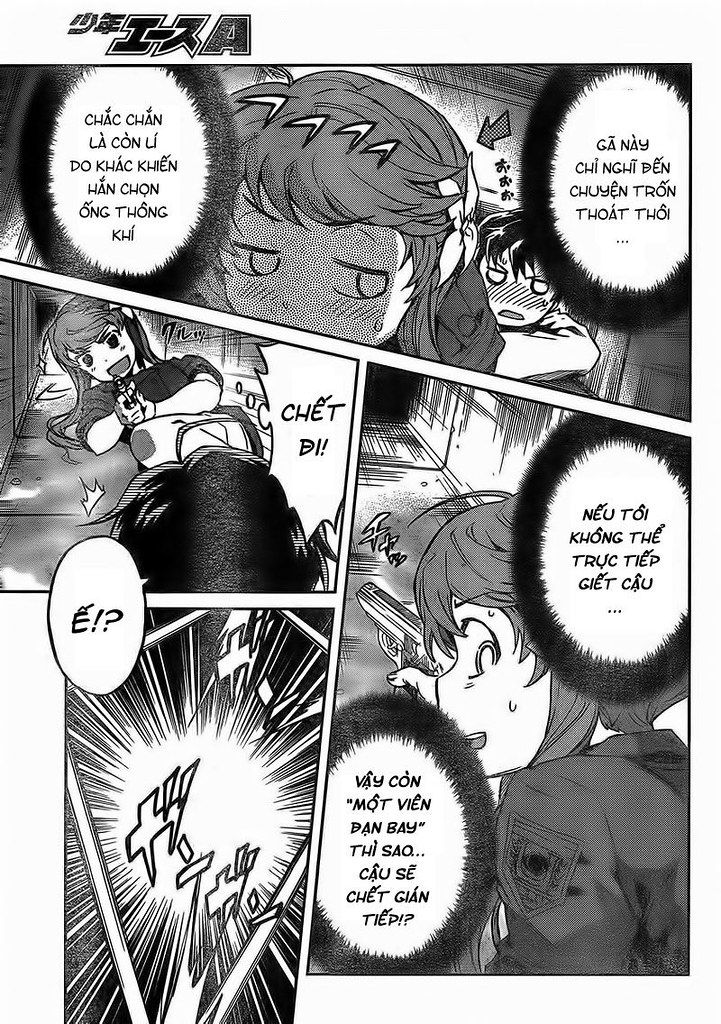The page from the comic book presents a tense, emotional scene rendered in black and white or grayscale, with four distinct panels. The top panel features a close-up of a crying girl, her face full of sorrow, contrasting with an angry boy in the background. Two speech bubbles, written in an unidentified foreign language, flank this image. 

In the second panel below, the girl is visibly tense, holding a gun pointed at an unseen figure turned away from the front. The third panel depicts dynamic explosion lines accompanied by foreign text, emphasizing action and heightened drama. 

The final panel to the bottom right shows the boy, now equipped with a gun, contributing to the escalating conflict hinted within the story. Two speech bubbles with foreign text float near him, adding depth to the intertwined narrative. The exact unfolding of events remains ambiguous due to the foreign language, potentially Asian, though not necessarily Japanese, and possibly Vietnamese.